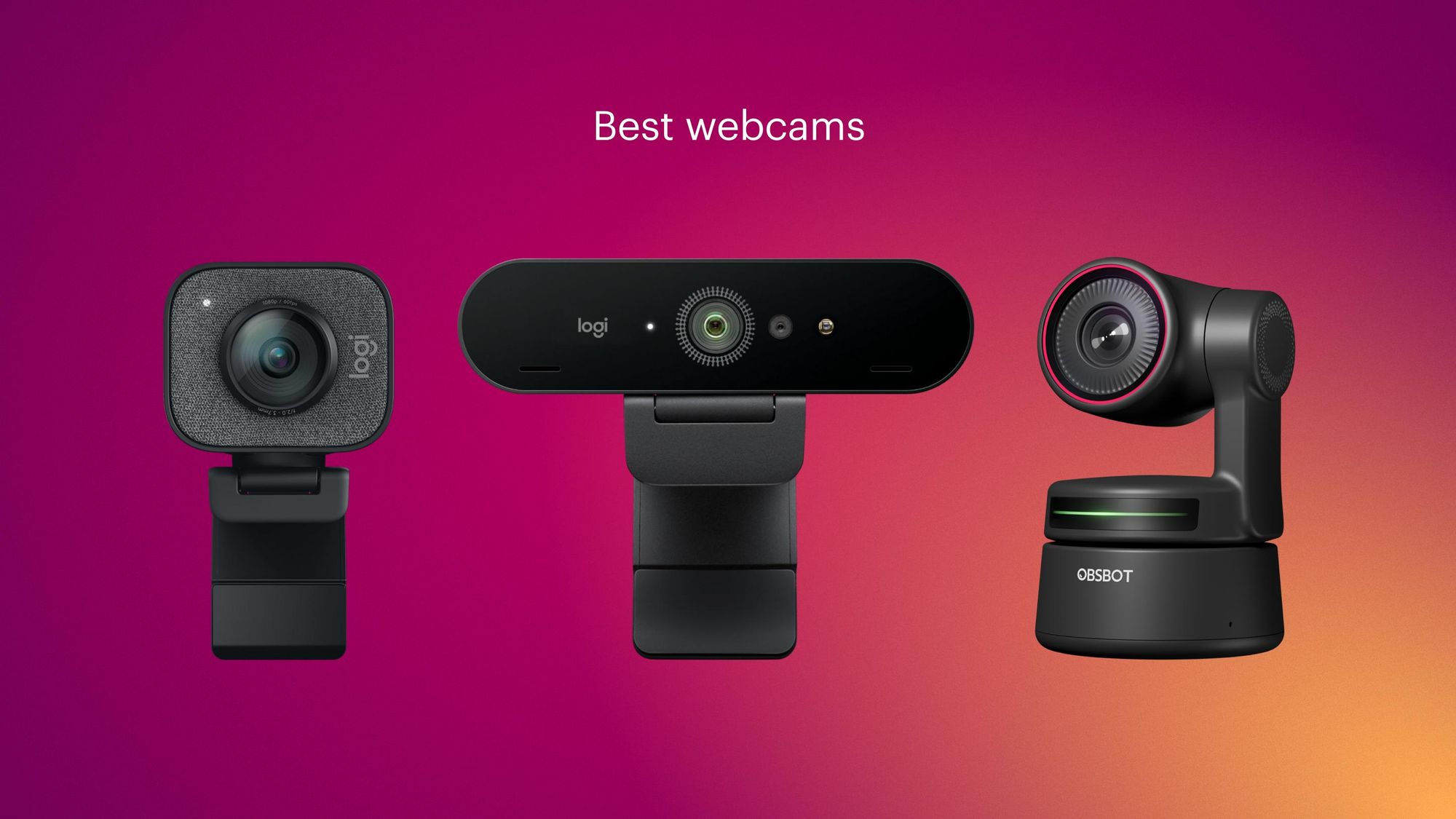This sales ad for Logie webcams features a striking ombre background that transitions from magenta-purple in the left corner to peach-orange in the right corner. At the top center, bold white text proclaims "Best Webcams." Below this caption, three distinct webcam models are showcased. 

The first webcam, positioned on the left, has a compact, rounded square design with a circular lens at its center. The body, reminiscent of a GoPro, has a black-and-white speckled texture and features the brand name "Logie" in white lettering on its side. It's mounted on a black bracket which allows for pivoting and rotation.

In the middle, the second webcam resembles a long oval with a rounded rectangular shape. Its main circular lens is flanked by additional small sensors and possibly a flash. The "Logie" brand is visible, and it too is affixed to a black stand that provides rotational capability.

The third webcam, on the right, stands out with a round base and a design that suggests it might be a 360-degree camera. It features a singular prominent lens bordered by a red ring and has a pivoting mechanism on its base. This model, like the others, prominently displays the "Logie" branding.

Together, these three webcams highlight the range and versatility of Logie's camera offerings against a vibrant, gradient backdrop.